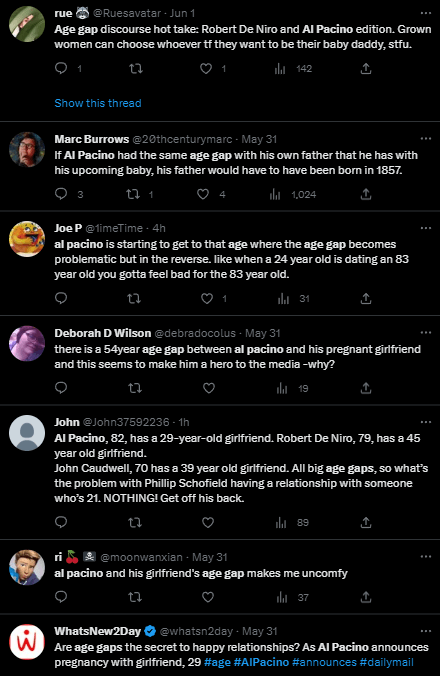In a lively conversation about age-gap relationships in Hollywood, several notable pairings were discussed. The debate kicked off with a fiery statement asserting that grown women have the right to choose any partner they want, regardless of age. This was followed by a humorous yet thought-provoking remark regarding Al Pacino, noting that if he had the same age gap with his own father as he does with his upcoming baby, his father would have had to be born in 1857.

Another participant, Joe, pointed out that while Al Pacino is reaching an age where significant age gaps often become problematic in reverse—like a 24-year-old dating an 83-year-old—it’s the elderly partner who might actually draw sympathy. Debra then highlighted the 54-year age gap between Al Pacino, 82, and his pregnant 29-year-old girlfriend, questioning why this makes him a hero in the media. She compared this to other significant age differences in celebrity relationships: Robert De Niro, 79, with his 45-year-old girlfriend, and John Caldwell, 70, with his 39-year-old girlfriend.

Debra concluded by questioning the criticism faced by Philip Schofield for his relationship with a 21-year-old, implying a double standard. She admitted that the age gap between Al Pacino and his girlfriend makes her uncomfortable.